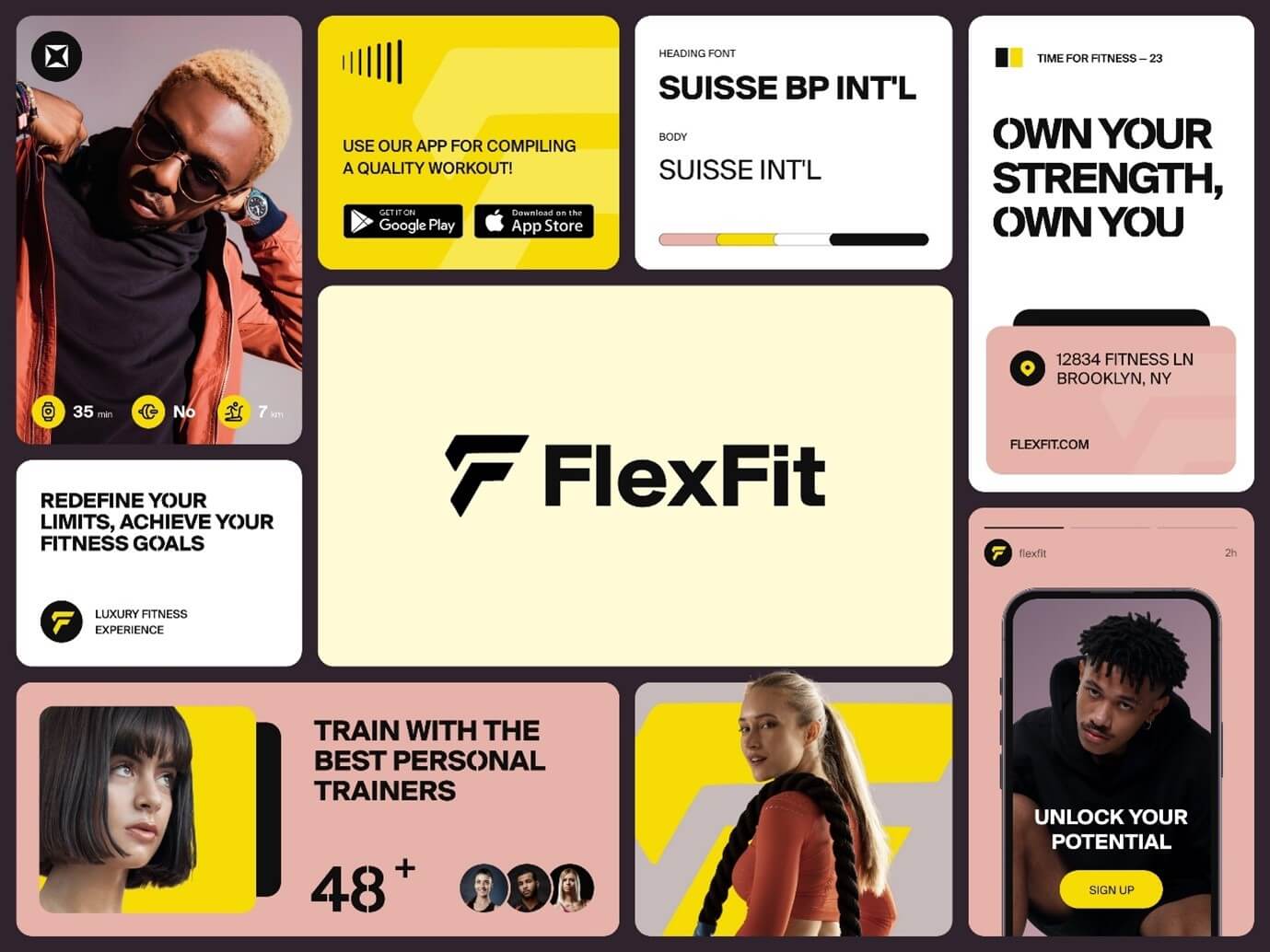The image is an advertisement for Flex Fit, prominently featuring a rectangular center block with a light yellowish-tan background, displaying the black "Flex Fit" logo, styled as an incomplete "F." The central message promotes the fitness app, available on Google Play and the Apple Store, with slogans like "Use our app for compiling a quality workout."

Around the central block, various smaller boxes showcase different promotional elements and pictures of people. In the top left corner, there's an image of a man in a hoodie, watch, and sunglasses, striking a casual pose. Below this, text encourages users to "redefine your level, your limits," and "achieve your fitness goals." 

The bottom right features a man in a sweatshirt and shorts looking directly at the viewer, with "unlock your potential" next to him. Adjacent to his left, a woman in workout attire is shown in profile, glancing back at the viewer with a battle rope over her left shoulder.

In the bottom left, there is a profile picture of a woman with a bob haircut, accompanied by the text "train with the best trainers, 48+," and images of three personal trainers. Additional ads around the perimeter include motivational messages like "own your strength, own you" and the gym's address, "12834 Fitness Lane, Brooklyn, New York," and their website, "flexfit.com." The color scheme features accents of yellow, black, tan, white, and salmon, reinforcing the energetic and motivational vibe of the advertisement.